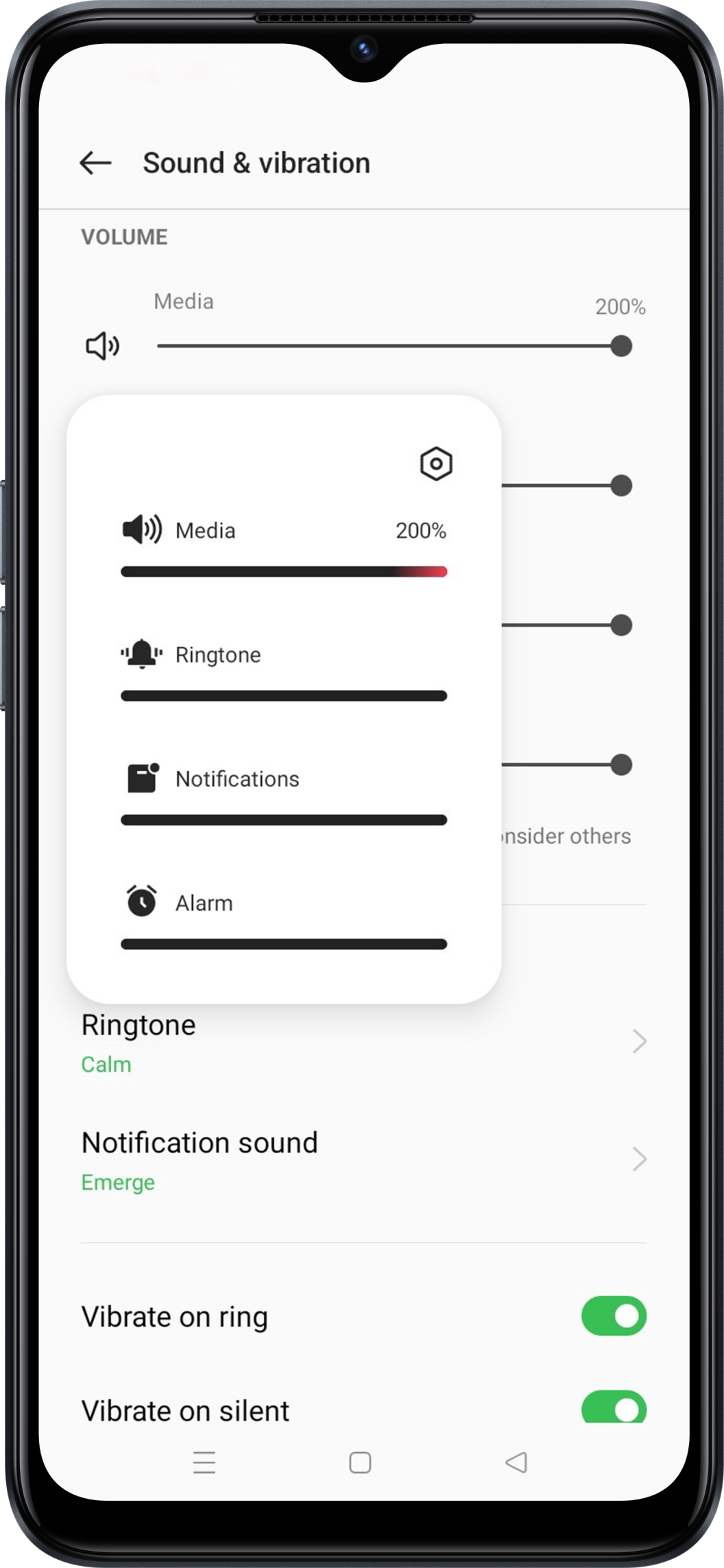The image is a photograph of a smartphone displaying its "Sound and Vibrations" settings. The phone's frame is visible, emphasizing that this is a captured photo rather than a direct screenshot. The background of the screen is white. In the upper left corner, "Sound and Vibrations" is written in dark gray font, accompanied by a left-pointing arrow.

Below this heading, the label "Volume" is visible, and a settings adjustment box is superimposed over the main interface. This box is predominantly white and square-shaped, detailing various volume levels—specifically for "Medium." Beneath the "Medium" label, the options "Ringtone," "Notification," and "Alarm" are listed sequentially, each separated by fine black lines.

Outside the settings box, the screen shows additional information. The "Ringtone" option indicates a choice labeled "Calm" in green text. Similarly, the "Notification" sound is set to "Emerge," also in green text. At the bottom of the display, the options "Vibrate on Ring" and "Vibrate on Silence" are both activated, as evidenced by the green oblong toggle switches on the right side of the screen.